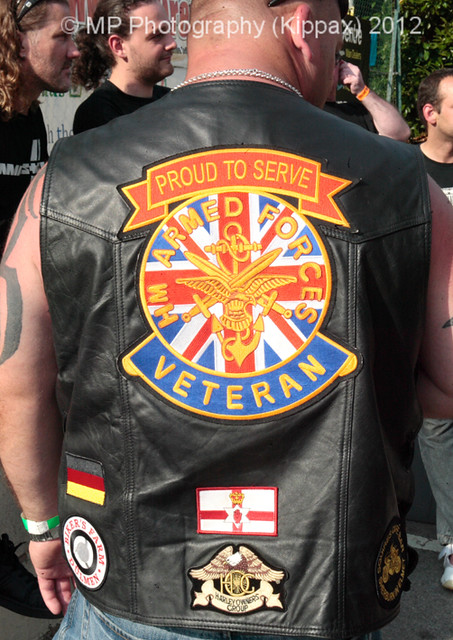In this close-up outdoor photograph by MP Photography (Kippax, 2012), the focal point is the back of a large, bald man wearing a sleeveless black leather jacket adorned with numerous patches. His jacket occupies the majority of the image, with the top of the jacket prominently displaying a red ribbon with gold lettering stating "Proud to Serve." Below this is a circular emblem with the text "H.M. Armed Forces" surrounding a gold, nautical-themed logo. Further down, a blue ribbon with gold lettering reads "Veteran." The bottom of the jacket features four patches, displaying various logos and flags, including a German flag. The man, who has a large build, sports a silver chain around his neck and has sunglasses perched atop his head. His upper left arm, visible in the image, is tattooed, and he is dressed in blue jeans. The background reveals trees, plant life, and people who are standing and facing to the right, adding context to the outdoor setting.